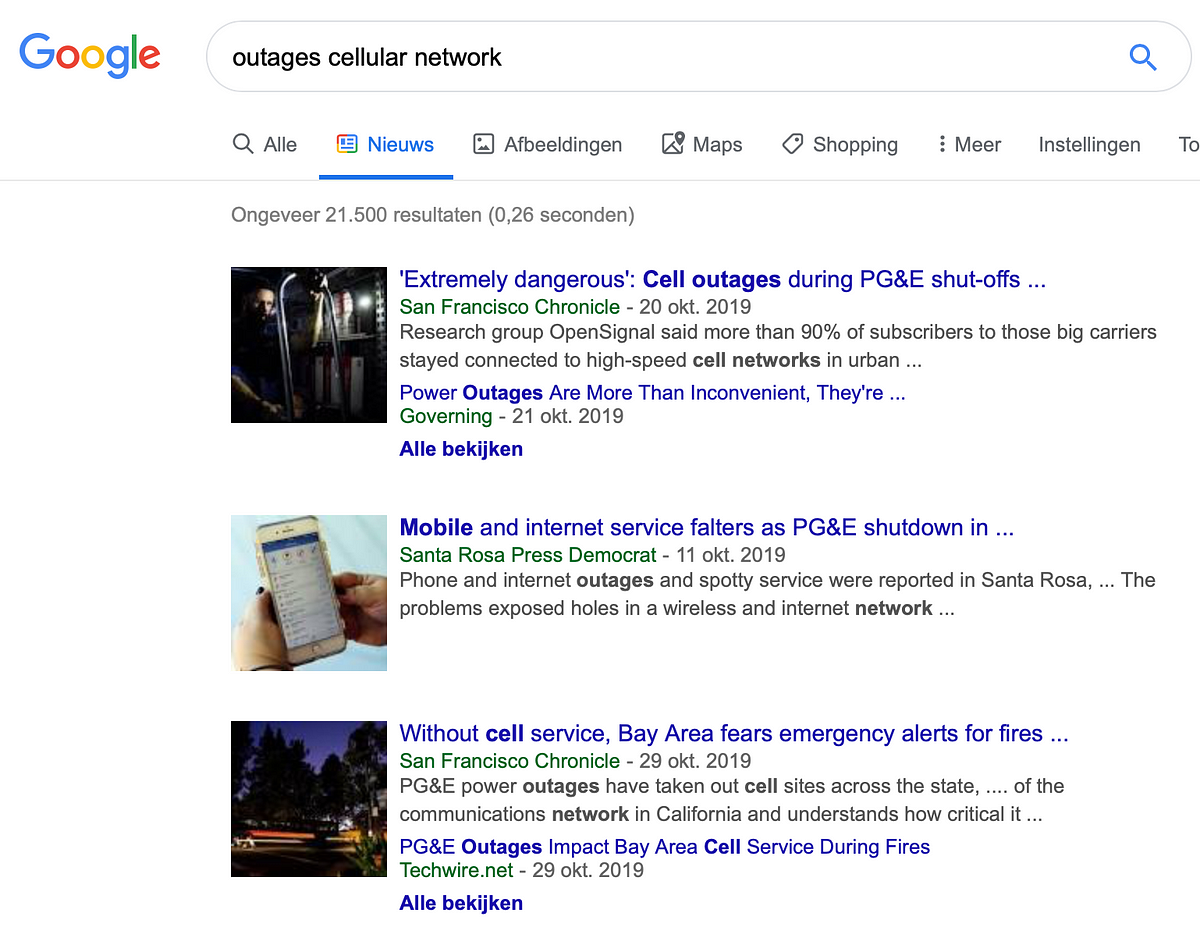This image is a screenshot of a Google search results page. The search query in the search bar reads "outages cellular network." The Google interface, including the menu bar and other UI elements, is in German, suggesting that the user is accessing a localized version of Google in a language other than English. The menu bar, featuring options in German, indicates that the user is currently viewing the "News" tab, evident from a blue-colored illustration resembling a newspaper with the word "Nachrichten" (which translates to "News") underlined, while the rest of the menu options remain in gray text, not bold or underlined.

The visible search results on the page are in English and display three news articles related to cellular network outages. The first article, sourced from the San Francisco Chronicle, is titled "Extremely dangerous cell outages during PG&E shutoffs." The second article, from the Santa Rosa Press Democrat, is titled "Mobile and Internet service falters as PG&E shutdown in...". The third result, also from the San Francisco Chronicle, is titled "Without cell service, Bay Area fears emergency alerts for fires...". These articles collectively highlight the pressing issue of cellular network outages during PG&E shutoffs, especially concerning emergency communications in the Bay Area.